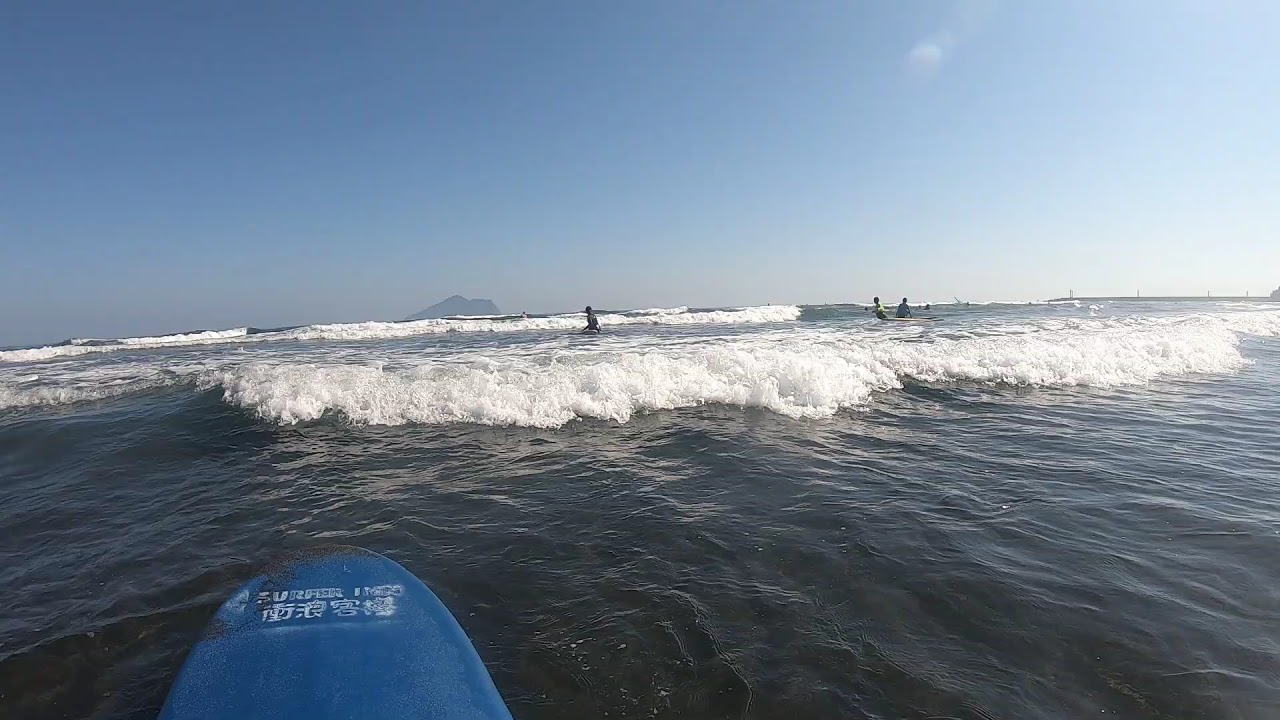In the vibrant image, we see the ocean basking under the bright, sunny sky, with clear, blue water reflecting the sun's rays. The perspective is from a blue surfboard marked with white Asian characters, suggesting that the photo might have been taken in an Asian country. The surfboard is aimed at incoming waves, highlighting the anticipation of an exhilarating ride. The waves, appearing distinct in two sets, create a dynamic scene – the closer wave has thick foam on its left and less on the right, while the farther wave has the opposite pattern. The ocean is a playground for several people, some surfing and others boogie boarding, scattered between the two waves. Despite a few clouds, the sky remains predominantly clear, adding to the idyllic setting of this picturesque day at the beach.